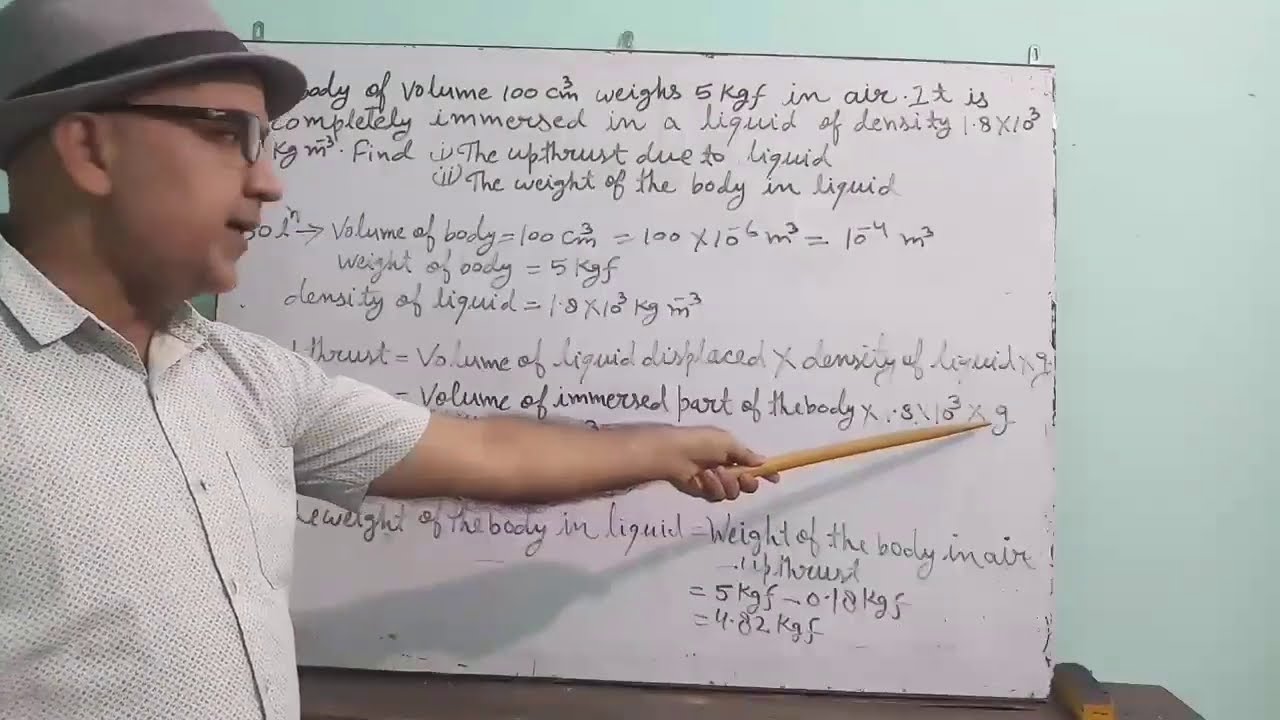The photograph captures a scene set indoors with a sea green backdrop. In the foreground, a man stands to the left side of the frame, occupying about a third of the image. He is a Caucasian gentleman wearing a short-sleeved, button-down shirt adorned with a small black and gray pattern. The shirt also features a pocket on the left breast. He sports black-rimmed glasses and a gray fedora with a black band around the brim, revealing a bald head. The man holds a classic wooden pointer stick in his left hand, directed at a whiteboard resting on a dark wooden table. The whiteboard is bordered in black and displays various equations written in cursive, pertaining to the densities and volumes of liquids. The man appears to be explaining a chemical process or calculation involving volume and liquid displacement, with the pointer targeting a specific part of the equation. His mouth is slightly open, as if caught mid-sentence, and his right eye is clearly visible due to the profile angle of the shot. The image quality ranges from poor to medium.